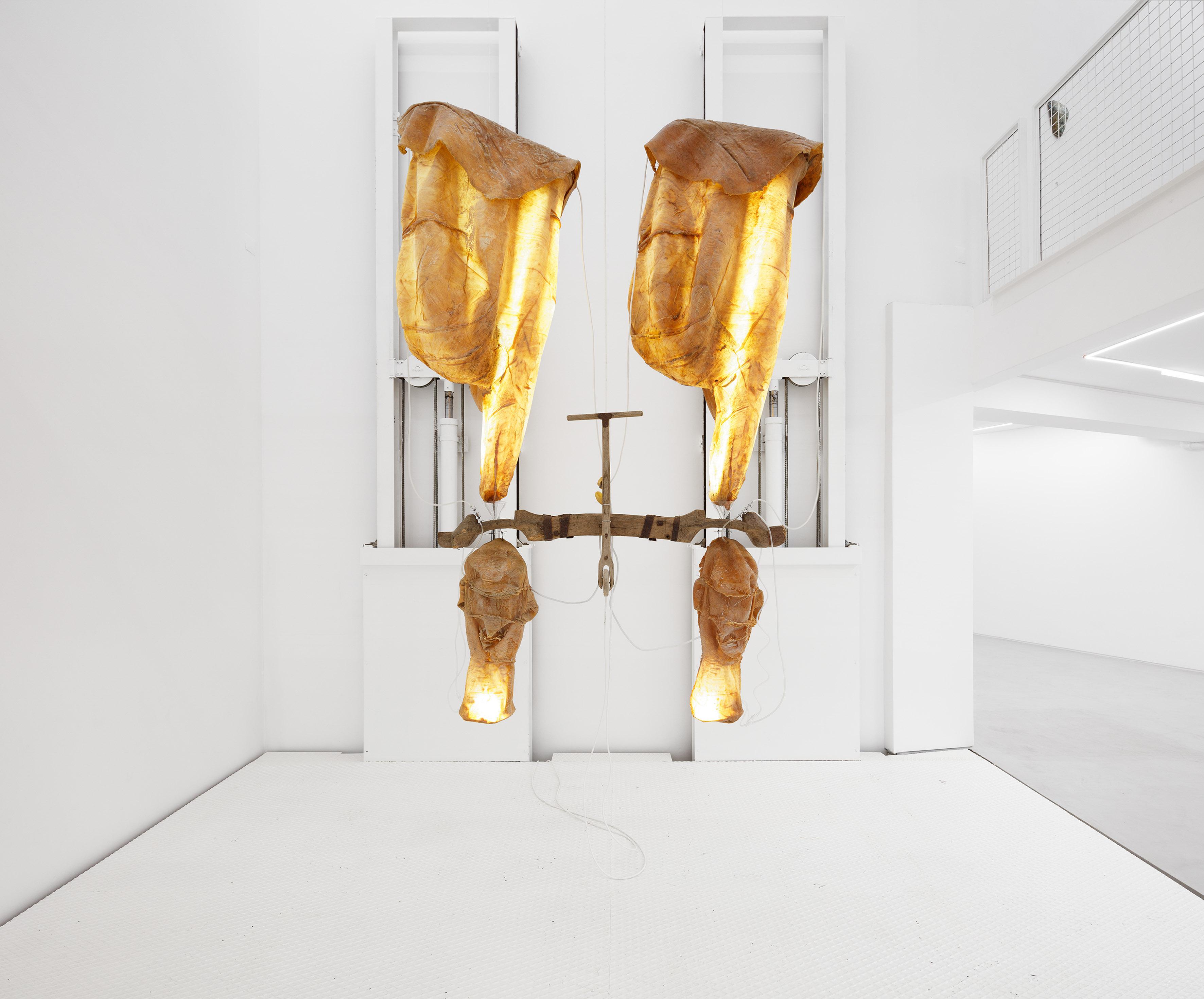The image depicts a perplexing modern art exhibit situated in a stark white museum gallery, with white walls, floors, and ceiling contributing to a highly illuminated space. The artwork consists of two identical structures, primarily golden in color with some brown and goldish-brown variegated fabric elements. Each structure is reminiscent of a bow, with additional components that evoke the appearance of internal organs or flesh, creating an unsettling impression. From the top of these structures hang what seem to be face-like masks or human heads, lending a more bizarre and thought-provoking aspect to the pieces. The exhibit is partially enclosed, with visible corners of the room enhancing the confined, introspective atmosphere. Despite its intended purpose to provoke thought, the exact nature and symbolism of the artwork remain ambiguous and abstract.